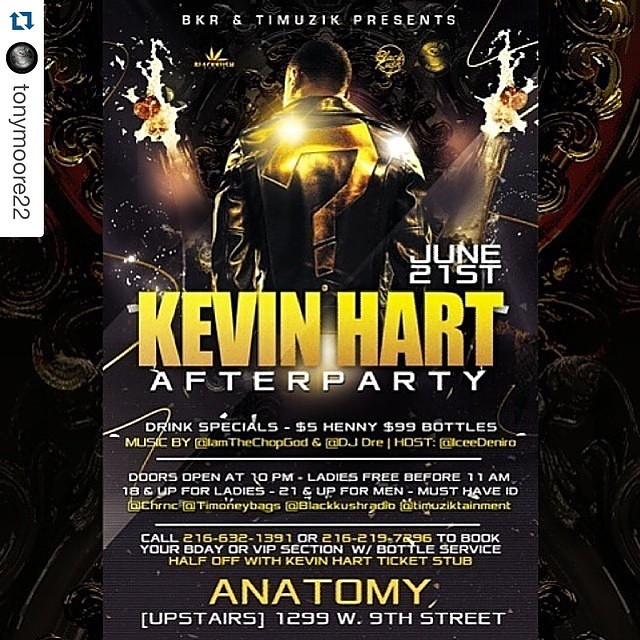The advertisement features a striking contrast with a black background that seems to swallow light, creating a stark, electrifying atmosphere. This dark backdrop accentuates vivid yellow and white lettering that almost glows, commanding attention and evoking a sense of energy and excitement. At the forefront is a dark-skinned figure with close-cut hair, depicted from the back wearing a black jacket adorned with a yellow question mark, adding a mysterious and powerful element that invites curiosity.

At the top of the poster, it states, "BKR and Tim Uzick presents" in white letters, alongside a round symbol and the name "Tony Moore 22." Beneath this, in large yellow letters, is the name "Kevin Hart," followed by the "After Party" text in white print. Below this, further details are provided, including the event date, "June 21st," and specifics about the event: drink specials ($5 Henny, $99 bottles), music by @iamtheChopGod and @DJDre, and hosting by @IcyDeNiro. The poster also indicates that doors open at 10 p.m., with ladies free before 11 a.m., noting age restrictions (18 and up for ladies, 21 and up for men) and a requirement for ID. Additionally, contact numbers are given for booking and VIP section reservations, highlighting a half-off offer with a Kevin Hart ticket stub.

The event is located at "Anatomy," upstairs at 1299 West 9th Street, creating an intriguing, electrified atmosphere that promises a night of excitement and energy.